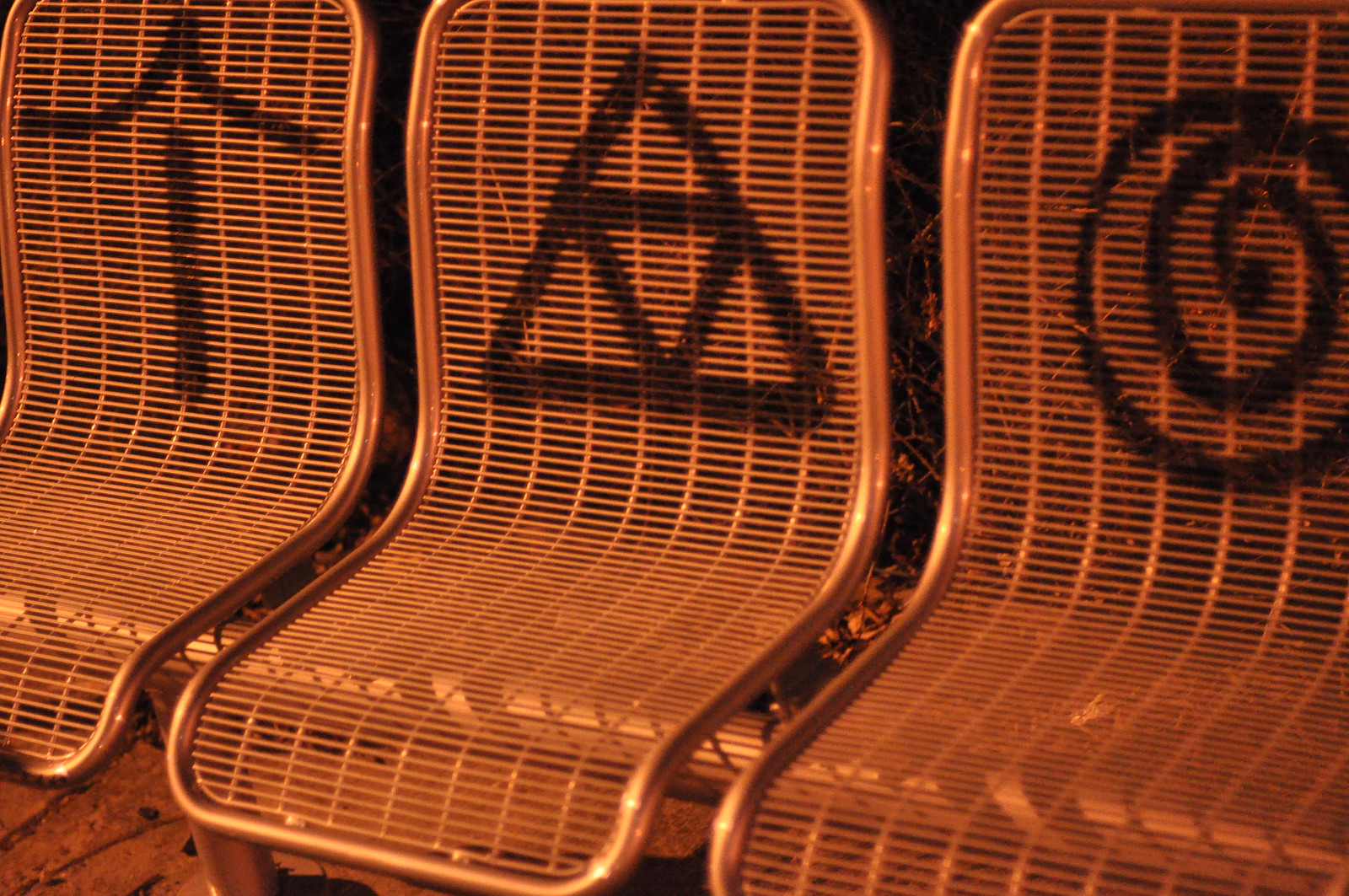The photograph captures a nighttime scene on a sidewalk illuminated by a street lamp, casting an orange glow over three metal chairs designed for public transport waiting, likely a bus stop. Each chair is constructed from high-quality metal with a vertical and horizontal grated design. There are clear spaces between the chair parts and no armrests, allowing for easy seating accessibility. Notably, each chair's backrest is adorned with distinct graffiti symbols: the first chair features a black spray-painted upward arrow, the second displays a black Triforce-like symbol consisting of a triangle with an upside-down triangle inside, and the third is marked by a black spiral or circular swirl pattern. The background shows some ground clutter, including scattered leaves, enhancing the urban atmosphere of the scene.